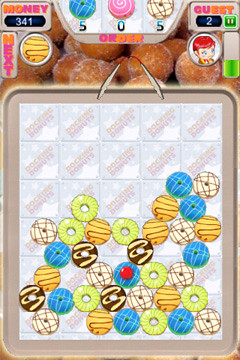Screenshot of a Mobile Game Interface: In the foreground, there is a virtual brown bag with a handle at the top, divided into multiple squared panels. Each panel houses a uniquely colored doughnut; some have holes in the middle, while others do not. The assortment includes lime green doughnuts, blue doughnuts, yellow and brown doughnuts, white and brown doughnuts, and dark brown and yellow doughnuts. The background features realistic photographs of doughnut holes, adding a layer of texture and depth to the image. In the top left corner, the word "Money" is displayed alongside an icon and a progress bar, indicating the player’s in-game currency. Similarly, in the top right corner, the word "Guest" appears with an accompanying icon and progress bar, likely signifying the player's guest status or progress in the game.